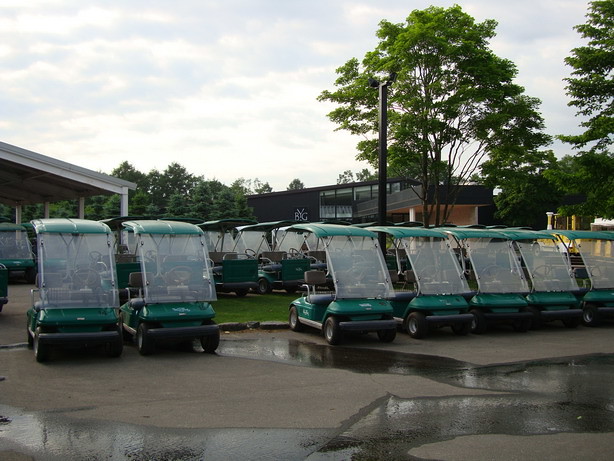In this overcast, natural light photograph, rows of emerald green golf carts are meticulously lined up in a parking lot, creating a striking visual of uniformity. Each cart features a slightly translucent Perspex windshield and black bumpers with side rails. The carts, boasting black tires with stainless steel silver circumferences, are parked in front of what appears to be a golf clubhouse. The ground is a light beige-brown concrete, dotted with large puddles of water. Behind the first row of golf carts, there is a green patch of grass, and towering, incredibly tall trees reach out of the frame on the right side. The sky is mostly overexposed with greyish-blue patches, adding to the moody atmosphere of the scene.